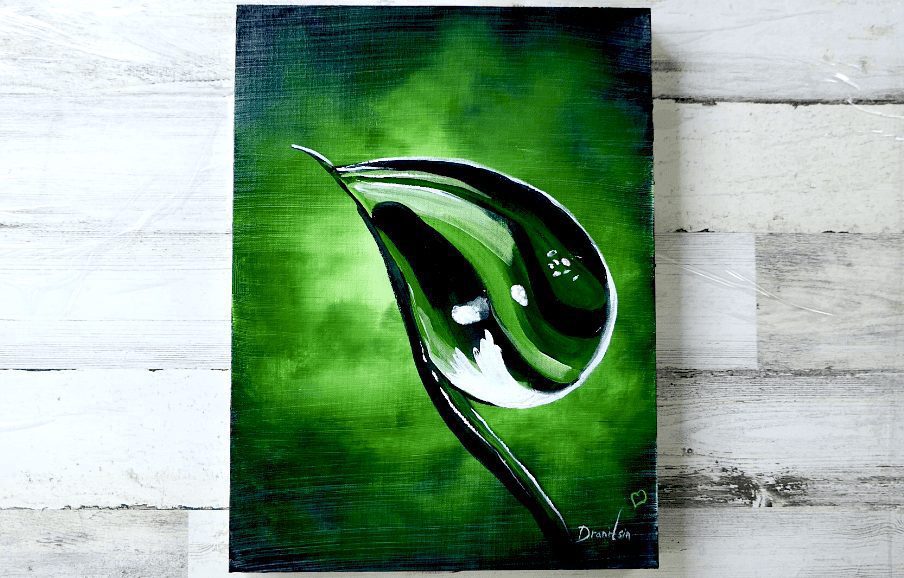This image showcases a detailed painting placed at the center of a white plank tabletop. The painting presents a striking contrast of colors, featuring a gradient that begins as a light, bright green at the center and transitions into a darker green and eventually black towards the edges, with a cloud-like texture that evokes the appearance of smoke. The focal point of the painting is a delicate water droplet perched on what appears to be the side profile of a leaf or a blade of grass. This droplet reflects the various green hues and hints of white, giving the impression of light bouncing off its surface. In the bottom right corner, the artist has signed the piece with a small white heart followed by the name "Dranlian." The overall tone of the artwork is abstract yet firmly rooted in nature themes, creating an alluring visual experience.